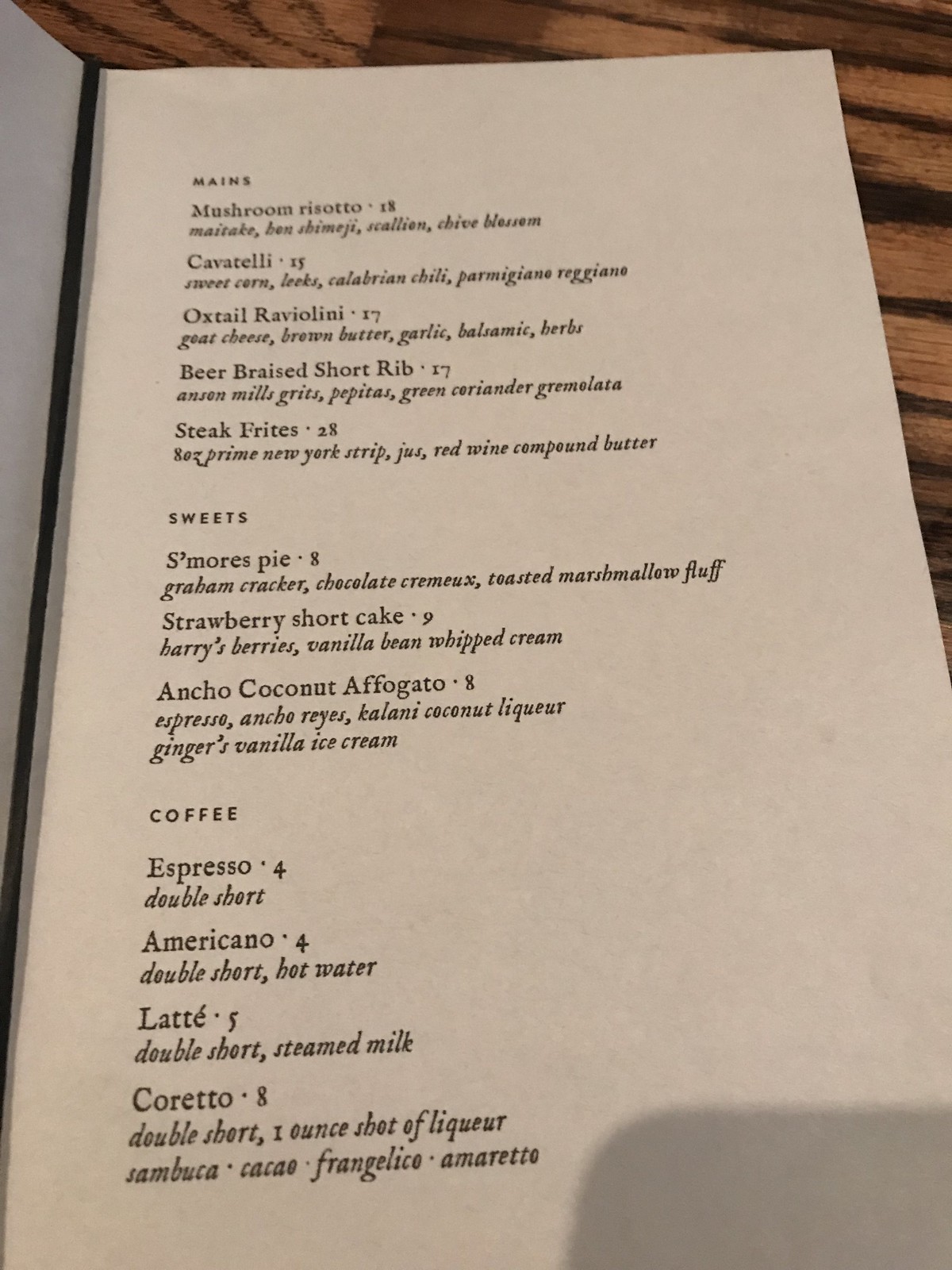This photograph captures a restaurant menu laid flat on a rustic oak wood table. In the bottom right corner, the shadow of the iPhone used to take the photo is visible. The menu is printed in black text and is divided into several sections. 

At the top, the section labeled "Mains" features:
- Mushroom Risotto, priced at $18
- Cavatelli, priced at $13
- Oxtail Raviolini, priced at $17
- Beer Braised Short Ribs, priced at $17
- Steak Frites, priced at $28

Each main dish is followed by detailed descriptions. 

Below the mains, the "Sweets" section lists:
- Schmorz Pie at $8, described with graham crackers, chocolate crèmeux, and toasted marshmallow fluff
- Strawberry Shortcake at $9
- Ancho Coconut Affogato at $8

At the bottom of the menu, the "Coffee" section offers:
- Espresso for $4
- Americano for $4
- Latte for $5
- Corretto for $8, specifically described as a double shot with one ounce of liqueur